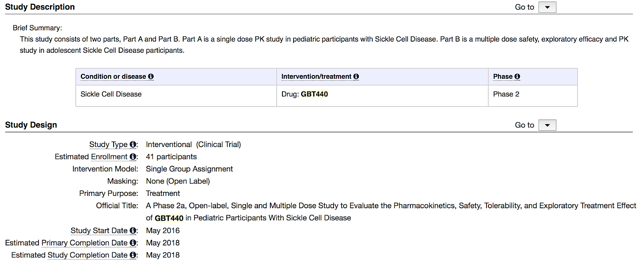The image features informational text centered around a study description. At the top, in bold black letters, the text reads "Study Description". To the right of this heading, there is a "Go To" dropdown menu button. A gray line extends horizontally below these elements, stretching from left to right.

Beneath the gray line, the text continues in non-bold black letters with "Brief Summary". This section explains that the study is divided into two parts: Part A is a single-dose pharmacokinetic (PK) study involving pediatric participants with sickle cell disease, while Part B is a multiple-dose safety, exploratory efficacy, and PK study targeting adolescent participants with sickle cell disease.

Directly below this summary, there is a light blue box that spans the width of the image, containing the text "Condition or Disease Intervention/Treatment Phase". 

Under this light blue box, there are three white boxes displayed side by side, labeled respectively from left to right as "Sickle Cell Disease", "Drug: GBT 440", and "Phase 2".

Further down in bold black letters is the heading "Study Design" accompanied by another "Go To" dropdown menu and a horizontal gray line beneath it. The descriptive text continues in non-bold black letters, indicating "Study Type: Interventional (Clinical Trial)" with an estimated enrollment of 41 participants.